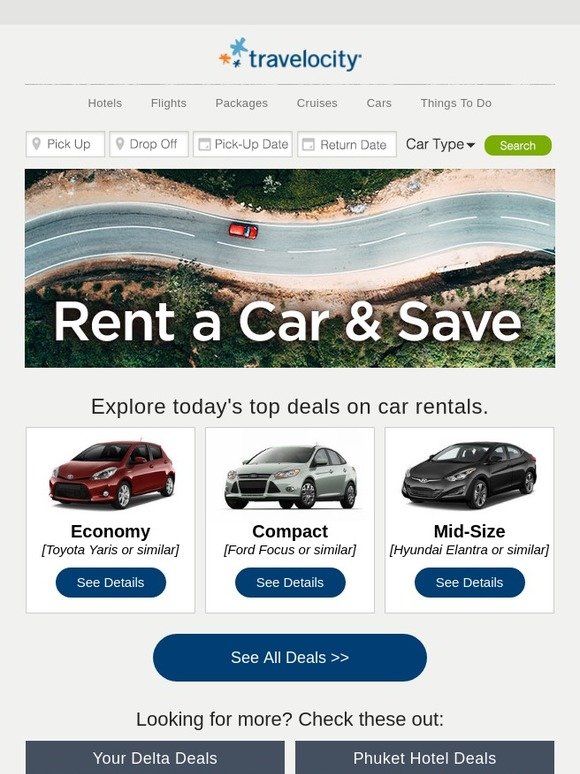This image captures a screenshot of the Travelocity website's car rental page. The top section features a gray background with the "Travelocity" logo prominently displayed in blue lowercase letters at the center. Below the logo, there's a faint horizontal line. Directly beneath this line is a navigation menu listing options from left to right: "Hotels," "Flights," "Packages," "Cruises," "Cars," and "Things to Do."

Further down, the interface includes four white selection boxes labeled: "Pick-up Location," "Drop-off Location," "Pick-up Date," and "Return Date." Adjacent to these, there is also a dropdown menu for selecting the "Car Type" and a prominent green "Search" button.

The main body of the screenshot features a large, captivating image of a red car navigating a curvy road. This is accompanied by the text "Rent a car and save," followed by the tagline "Explore today's top deals on car rentals."

Underneath the promotional image are thumbnails of three types of cars available for rental:
1. A red Toyota listed as an Economy vehicle.
2. A compact Ford Focus.
3. A midsize Hyundai.

Each car thumbnail includes a blue "See Details" button beneath it. At the bottom of these images, there is a larger button labeled "See All Details." Lastly, the page suggests additional options with the phrase "Looking for more? Check these out."